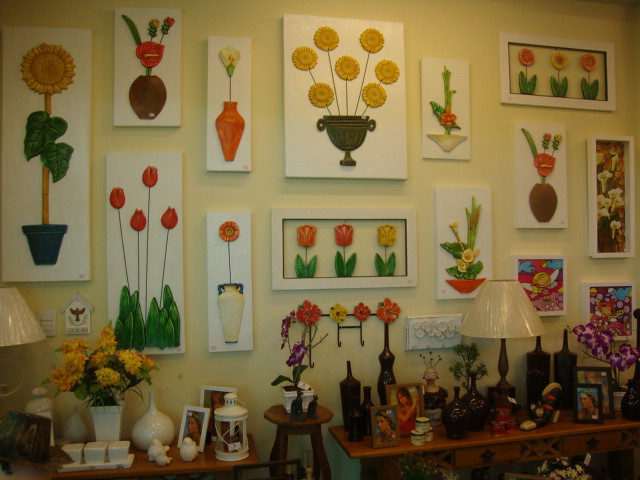The photograph captures a room with a creamy yellow wall adorned with 14 to 15 pieces of flower-themed wall art, mostly canvas paintings seemingly done in watercolors. These vibrant paintings depict various flowers in hues of red, yellow, orange, and green. Some of the art illustrates sunflowers, tulips, and daisies, exhibiting a detailed and illustrative style. Below the wall art, the floor hosts two wooden tables, one on the left and one on the right, each adorned with an assortment of items including picture frames—some containing repetitive photos that appear to be placeholder images—vases, flower pots, empty wine bottles, and decorative knickknacks. Between the tables stands a four-legged stool with a flower pot and plant placed on it. The scene is bathed in soft lighting from the lamps on the tables, enhancing the cozy, personalized ambiance of the room.